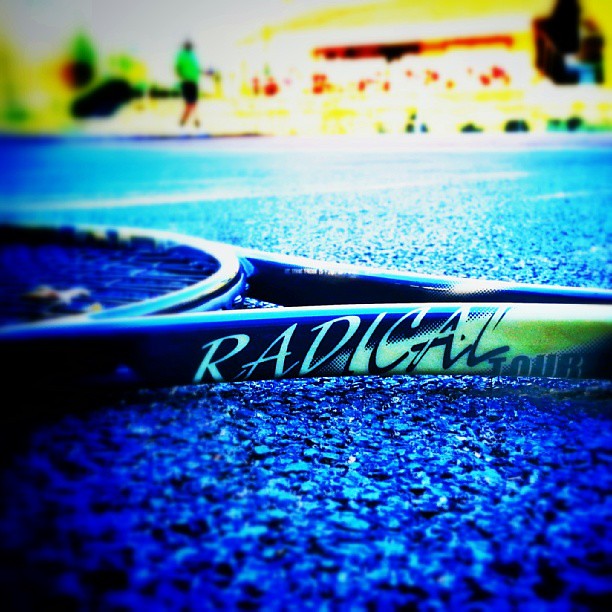This artistic photograph captures a tennis racket, titled "Radical Tour," lying on its side on the shockingly vivid blue surface of a tennis court. The image is taken from an almost ground-level perspective, highlighting the intricate texture of the court. The racket's 1980s-style lettering and netting are clearly in focus, making it the central element of the composition. In the distant, blurred background, you can discern an individual in black shorts and a neon green top walking on the court, lending a sense of activity to the scene. The backdrop also features a building, possibly a spectator seating area, though it remains indistinct due to the image's intentional out-of-focus technique. The overall color palette of the photograph is distorted, with a fluorescent, almost surreal blue and green glow dominating the scene.